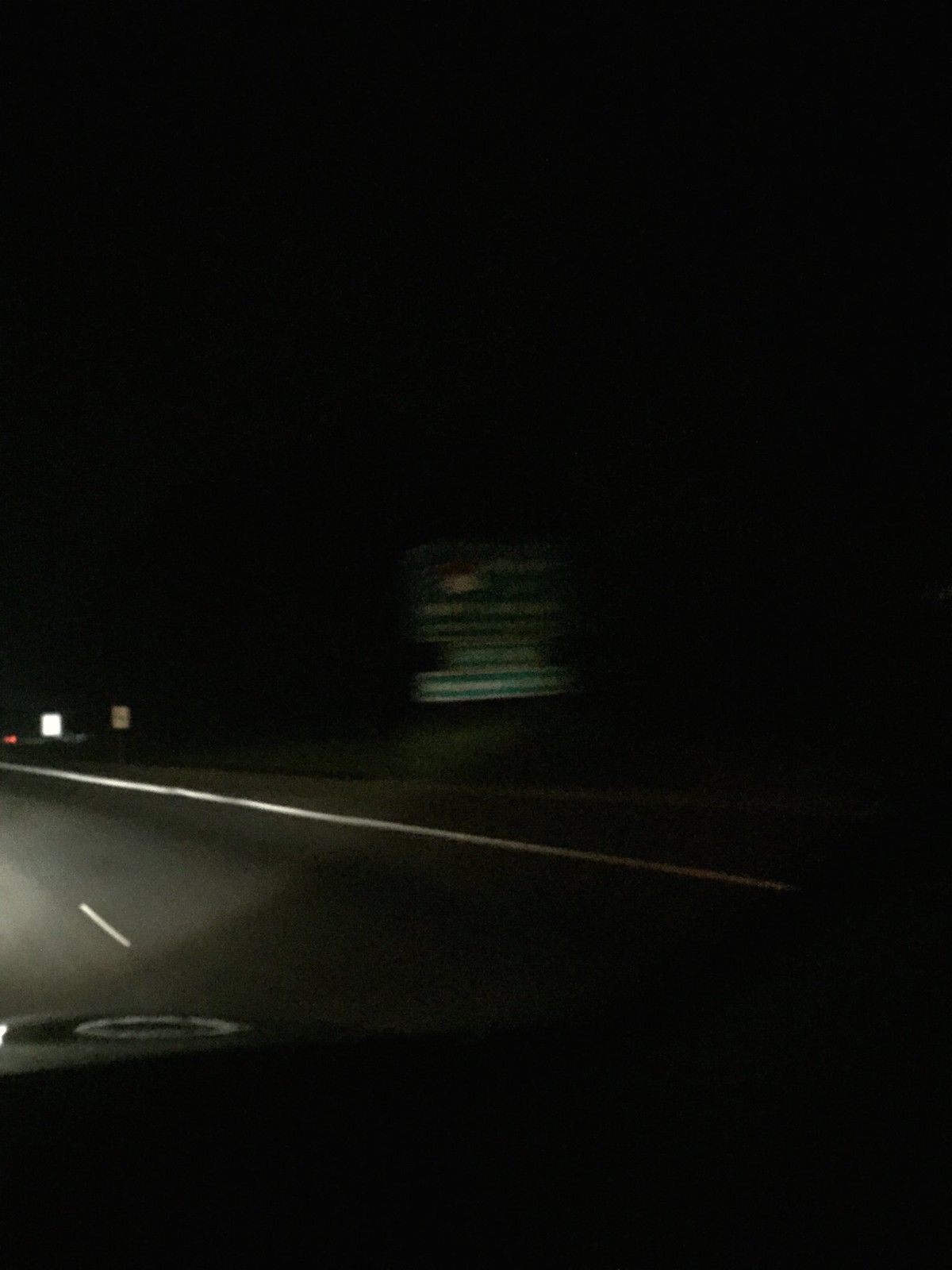Captured from a moving vehicle at night, this slightly vertical image illustrates a scene illuminated solely by the automobile's headlights. The picture focuses on a multi-lane interstate, distinctly showing the white line demarcating the edge of the right-hand lane, extending from just below the center right to the center left of the frame. Positioned near the center left of the image, a small speed limit sign is faintly visible. Towards the upper center, a green sign with white lettering—likely indicating an approaching exit—appears blurred and poorly lit, rendering its text unreadable. The vehicle's headlights reveal that it occupies the lane adjacent to the right-hand lane on the road.